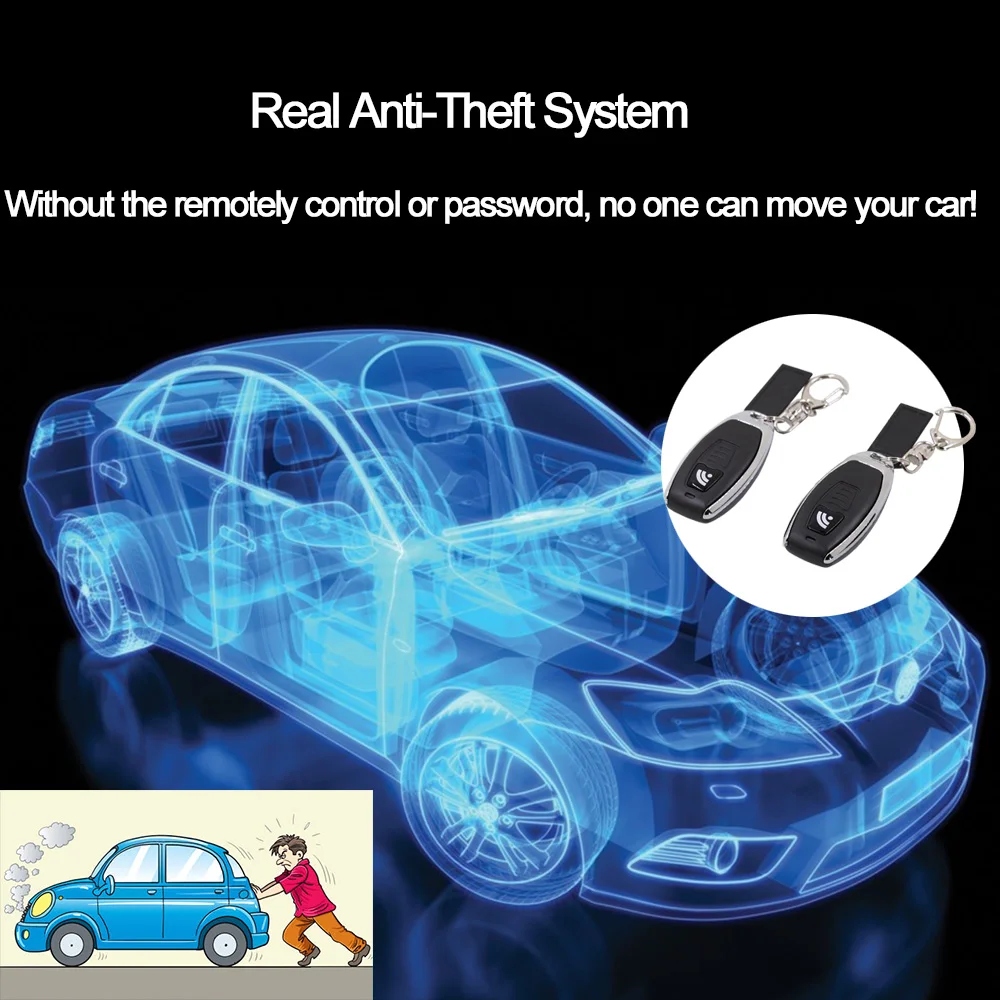This advertisement for a car anti-theft system features a black background highlighting a blue, x-ray-like transparent computerized diagram of a car. The top of the image prominently displays a banner reading, "Real Anti-Theft System. Without the remote control or password, no one can move your car." To the right, a white circle showcases two black and silver keychain remote controls, positioned at a three-quarters angle, likely in a showroom setting. At the bottom left corner, a cartoon depicts an angry man in a red shirt and brown pants huffing and puffing while pushing a struggling blue beetle car with smoke billowing from its hood, emphasizing the importance of the anti-theft system in preventing unauthorized vehicle movement.